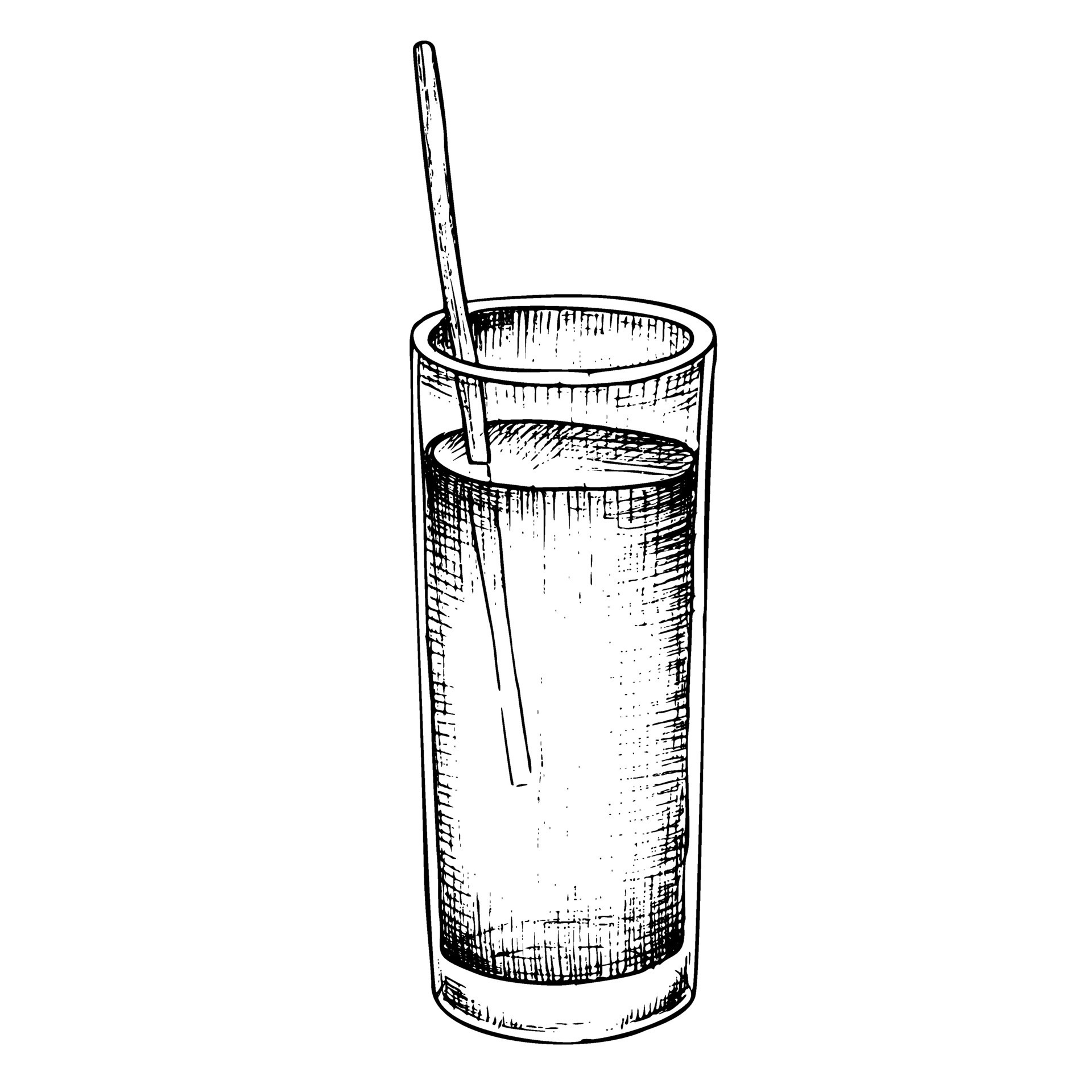This black and white illustration features a simplistic yet detailed line drawing of a tall, narrow, cylindrical glass filled with a liquid, likely water. The glass is depicted against a plain white background and is intricately shaded using a crosshatch technique to imply the presence of the liquid inside. The glass has a distinct rim at the top and appears to have thicker sides and bottom, adding to its structure. A straight straw, placed on the left side of the glass, extends about two-thirds into the liquid and protrudes upward an equivalent length above it, slightly tilting to the left. The artwork is devoid of any artist's signature or additional elements, focusing solely on the detailed portrayal of the glass and straw.